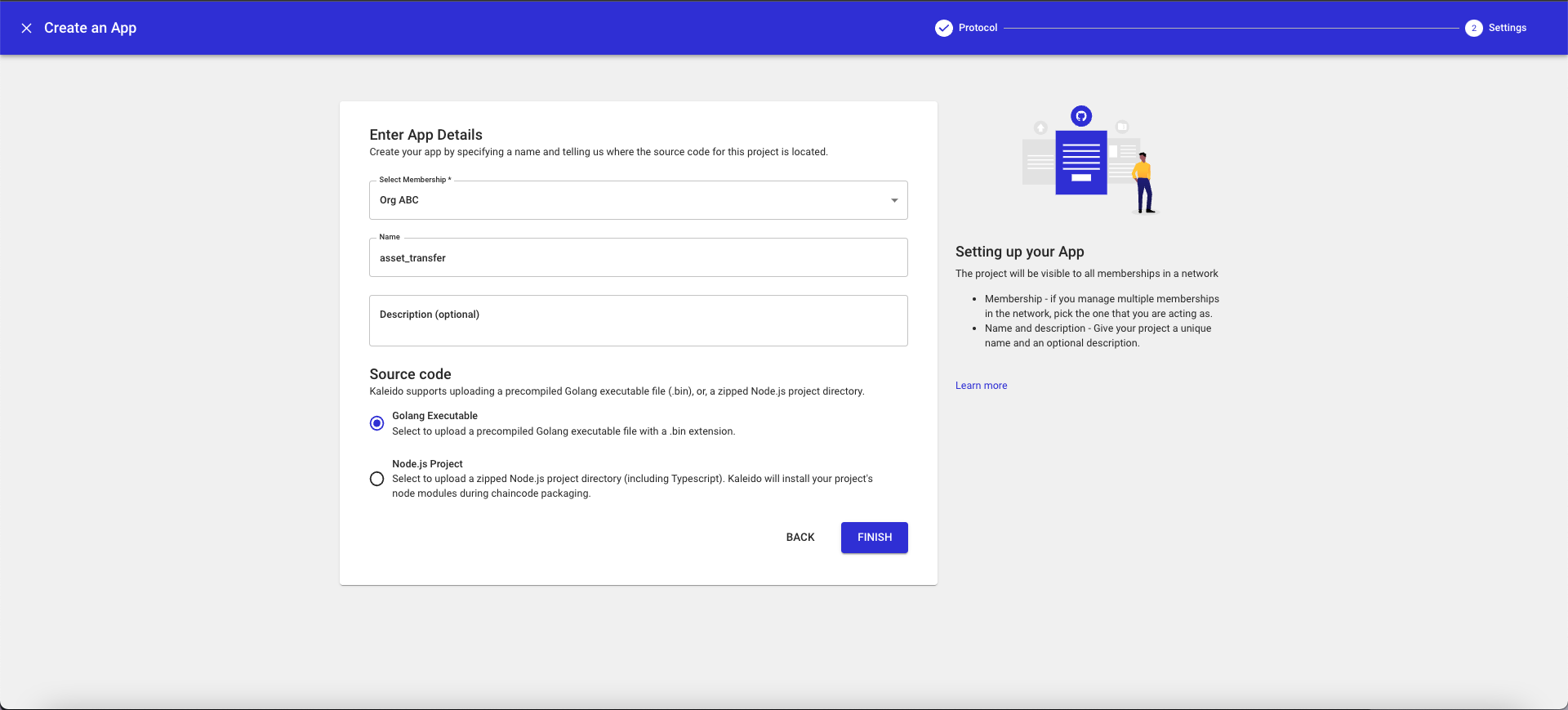This image captures a screenshot of a computer screen displaying an application creation interface. At the top of the screen, in a blue rectangle, a navigation bar is visible. On the left, there is an "X" labeled "Create an App." Toward the right of this bar, a checkmark is positioned next to the word "Protocol," followed by the text "Settings" next to the number "2."

Dominating the center of the screen is a large gray popup window titled "Enter App Details." The window prompts the user to "Create your app by specifying a name and telling us where the source code for this project is located." Under "Select Membership," the user has chosen "org ABC." The "Name" field is filled in with "asset_transfer," and the "Description" field is marked as "Optional."

At the bottom of the gray popup, under the "Source Code" section, instructions and options for source file formats are provided: "Kaleido supports uploading a precompiled Golang executable file .bin or a zip Node.js project directory." Two clickable options are available: "Golang executable" or "Node.js project." The user has selected the "Golang executable" option.

On the right side of the screenshot, an illustration shows a person near a page, accompanied by text reading "Setting up your app." The overall layout is clean and user-friendly, guiding users through the necessary steps to configure their application details effectively.